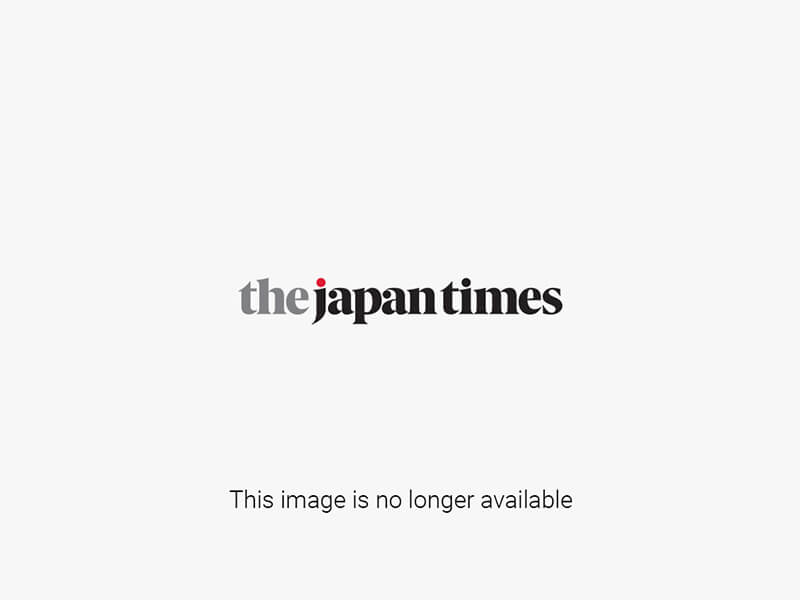This detailed color photograph, taken at the Kyocera Dome in Osaka during the Oryx Buffaloes championship game, captures the electric atmosphere of an overflow crowd of passionate baseball fans. The image, oriented in landscape, primarily features tightly packed spectators, predominantly East Asian with black hair, all fervently cheering and looking up to the right. Amid the sea of people, blue vertical rails angle across the stands, adorned with white vinyl underneath. Fans, some of whom are standing and clapping, proudly wear white jerseys emblazoned with "Buffaloes" and other Asian lettering, while a few don face masks. Concession stand vendors navigate through the densely populated rows filled with enthusiastic supporters. The photograph, rendered in a realistic and representational style, effectively conveys the vibrant and lively spirit of the fans from top to bottom of the frame.